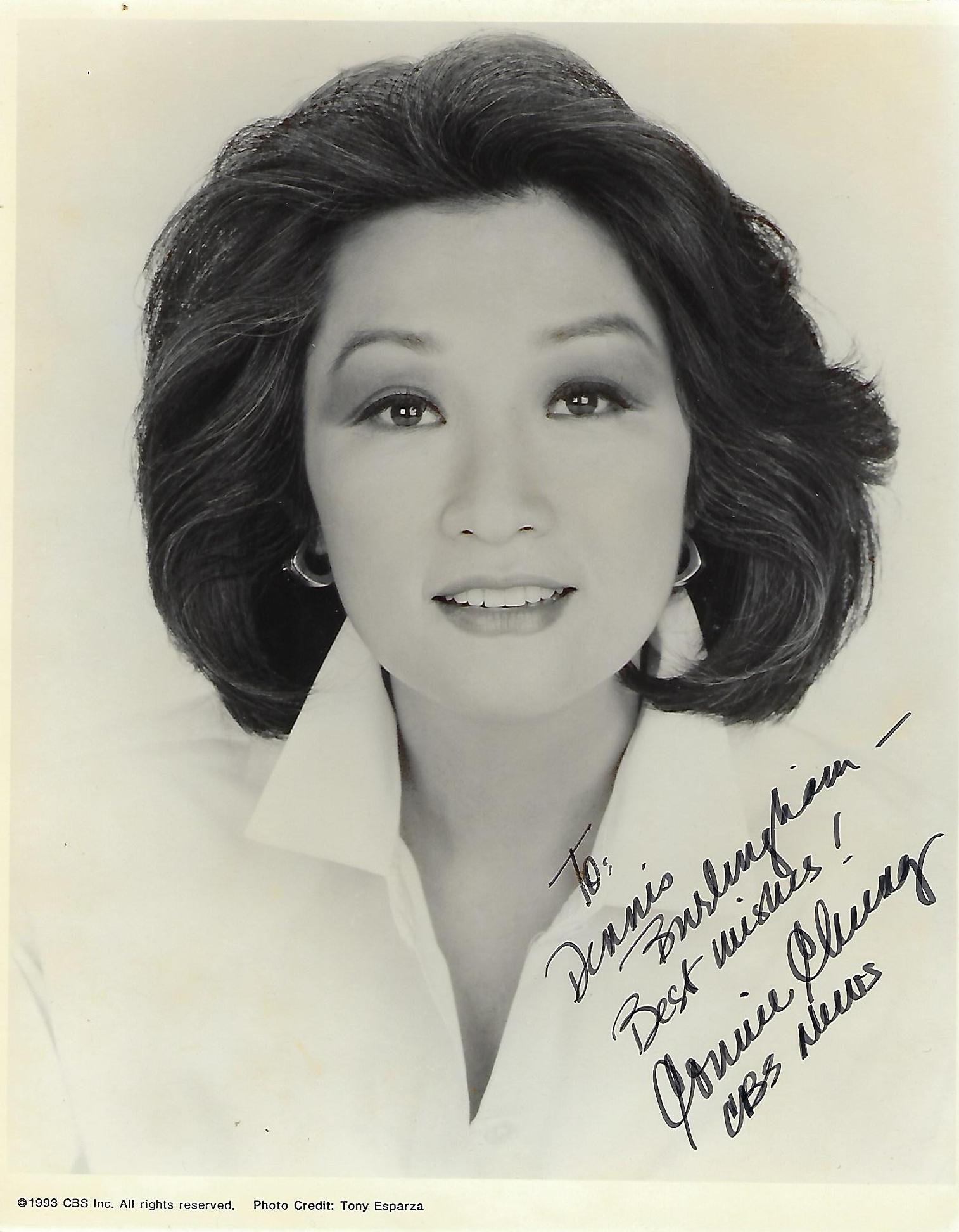This image is a black and white scan of a photograph featuring Connie Chung, taken in 1993 and credited to photographer Tony Esparza. The photograph shows Connie Chung wearing a white collared shirt and round earrings, with her wavy, dark hair styled shoulder-length. She appears to be wearing lipstick and looking directly at the camera against a slightly off-white backdrop. The image is personally autographed by Connie Chung with the inscription, "To Dennis, Best Wishes! Connie Chung, CBS News," written in black handwritten lettering on the bottom right side. Additionally, the text at the bottom left corner reads, "1993, CBS Inc., All Rights Reserved."